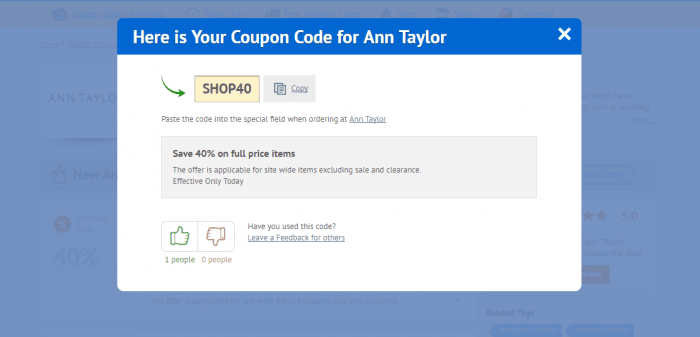Screenshot of an Ann Taylor promotional popup displaying a coupon code. The code is prominently featured alongside a small green arrow pointing to "Shop 40," which indicates a 40% discount on full-priced items. Users can easily copy the code and paste it into the appropriate field during checkout to avail the discount. The popup includes an exit 'X' icon on the top-right corner for closing the window. At both the top and bottom of the popup are like/dislike buttons allowing users to provide feedback on the coupon. The background is semi-transparent, adorned with stars, and prominently features the Ann Taylor logo. The text "Save 40%" is highlighted within a grey box, reinforcing the discount offer.